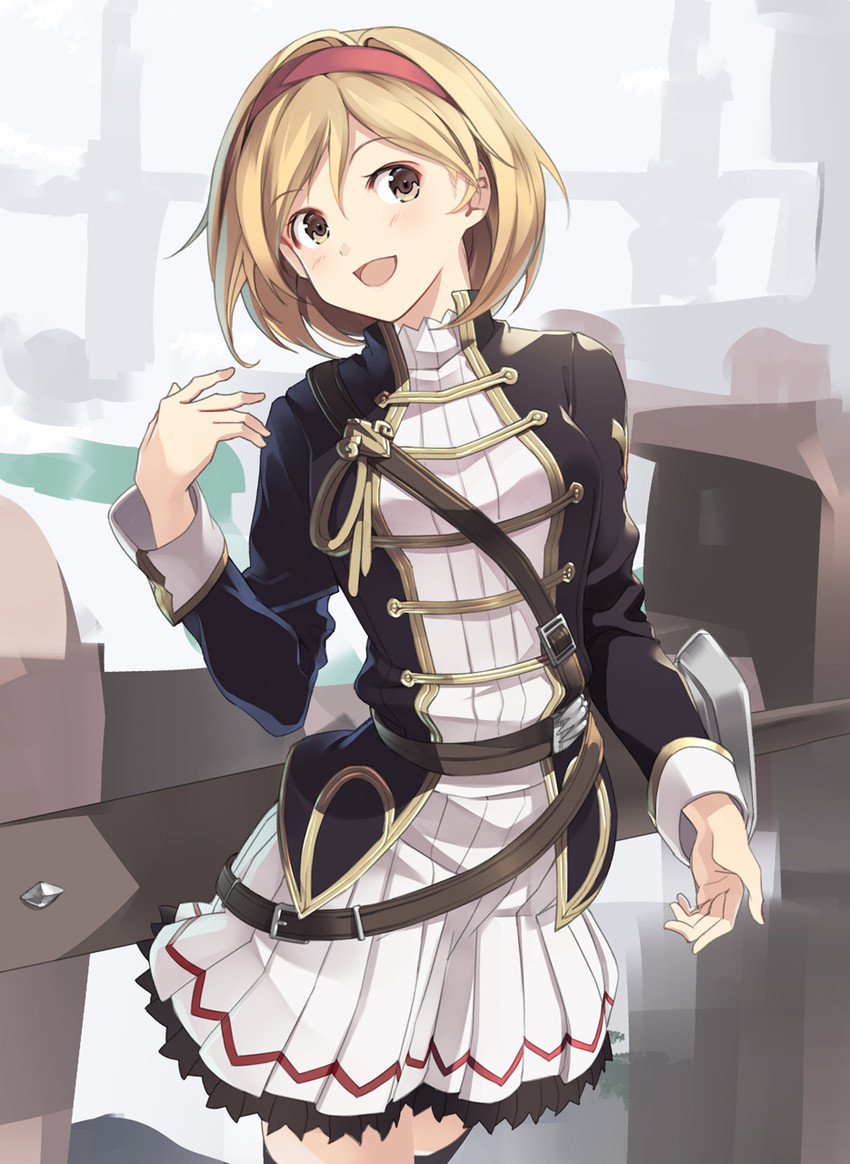This anime illustration features a young woman with chin-length, honey blonde hair, adorned with a red headband. Her head is tilted toward her right shoulder, and she possesses expressive light brown eyes with her mouth slightly open. She is dressed in a meticulously detailed black jacket that flares out at the waist, featuring gold piping and white cuffs accented with gold. Gold straps cross the front of the jacket, reminiscent of a Victorian-era or Napoleonic vest. Underneath, she wears a white dress with a short, pleated, and flared skirt, decorated with black and red accents, including a distinctive zigzag pattern around the bottom. Her outfit is further accessorized with several belts at different levels around her torso and waist, suggesting a blend of historical and fantastical elements. Although the background is vague and abstract, with indistinct lines and shapes, the character is illuminated by light, and she stands in front of what appears to be a partially visible vehicle or possibly a large, undefined object, adding a sense of mystery to the scene.